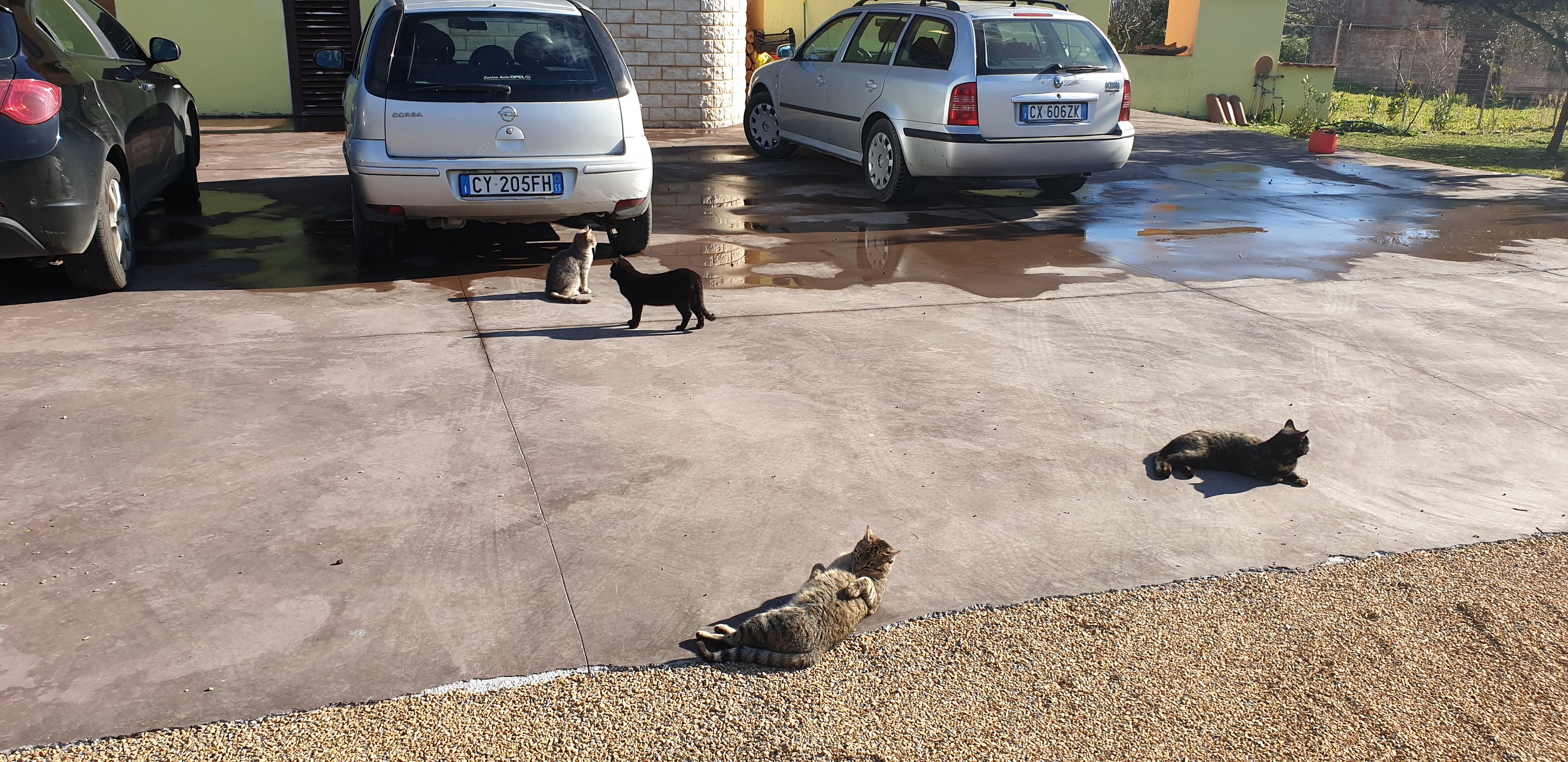This is a color photograph of an outdoor driveway or parking area, depicting a slightly wet ground surface composed of dark gray and large concrete tiles, bordered by a small gravel area. The scene includes three parked cars: a partially visible black car on the left, a grey car in the middle, and a station wagon-type grey car on the right. The driveway ground near the cars appears wet, possibly from recent washing, while the surrounding areas are dry. In the foreground and mid-ground, four cats are present—two are lounging on the ground in the sun, soaking up the rays, one grey cat is sitting upright, and another black cat is standing and looking at the sitting grey one. The background features a greenish building wall with a combination of white painted brick and light green concrete. There is also a visible EU license plate, suggesting a European locale. In the upper left-hand corner, some greenery is barely discernible, possibly indicating a yard or garden area. Additional elements include an orange pot and some grass, adding more life to this tranquil domestic scene.